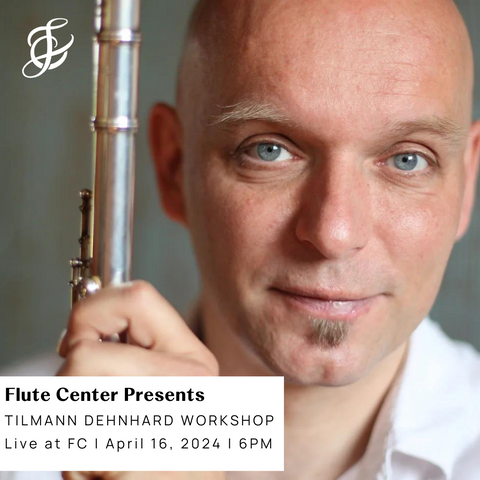This is a detailed promotional photograph featuring a bald man with bluish-gray eyes and thin, hard-to-see eyebrows. He has a distinct, small patch of facial hair just under his bottom lip, while his chin is clean-shaven. The image portrays him holding a silver-colored flute, suggesting a musical theme. He is dressed in a white collared shirt and exhibits a pleasant, cheery expression, with the light source illuminating him from the right side, casting shadows to the left. The background is grey, providing a neutral backdrop that highlights the subject. The photograph is overlaid with promotional text at the bottom left, reading "Flute Center Presents Tilghman Denard Workshop, Live at FC, April 16, 2024, 6 p.m." Additionally, the man's initials are positioned in the top left-hand corner, possibly rendered in intertwining text forming an "L" and a "C." The overall composition is square-shaped or slightly taller than it is wide, enhancing the prominence of the subject and the flute in his hand.